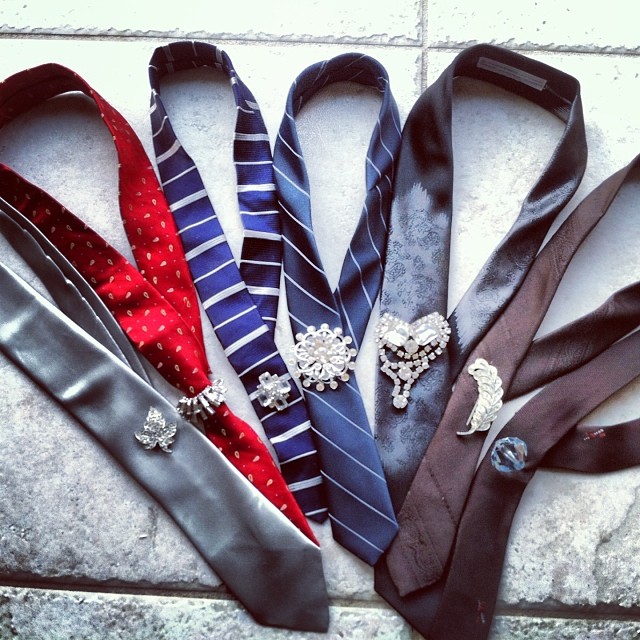This photograph captures six neatly arranged neckties laid out in an arched formation on a light gray stone tile floor. The tiles have dark gray edges and visible grout lines, adding texture to the background. From left to right, the neckties are as follows: 

- A silver-gray tie adorned with a diamond-studded maple leaf emblem. 
- A red tie featuring white spots and a silver circular pendant.
- A blue tie with alternating thick and thin horizontal white stripes, decorated with a chrome pendant.
- A darker blue tie with diagonal white stripes and a sailor's wheel emblem encrusted with diamonds.
- A gray tie with a heart-shaped pendant at the top narrowing into a long design at the bottom, studded with diamonds.
- A brown tie with a silver leaf-shaped clasp.

Each tie is elegantly pinned or clipped with a piece of jewelry, either diamond-encrusted or silver, adding a touch of sophistication to the display.